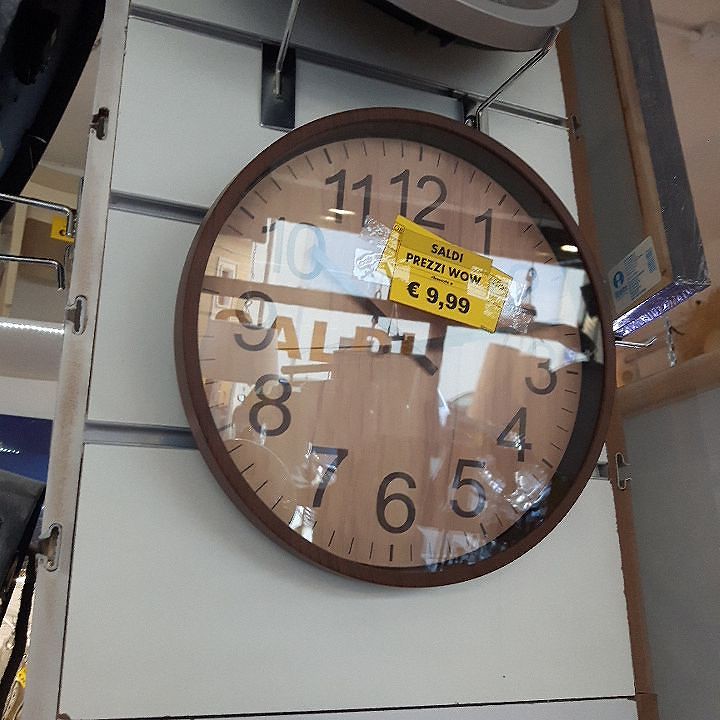This photograph captures a clock prominently displayed on a wall section within a store. The clock is mounted on a cabinet or display structure using wire hangers protruding from horizontal silver lines on the wall. The timepiece itself is circular with a brown edge, likely made of plastic, though it could also be glass due to its highly reflective and shiny surface. The reflections on the clock indicate it’s a sunny day, with sunlight streaming in from somewhere across the room. Within these reflections, the letters "C, A, L, R, I" or possibly "D, I" are discernible.

The clock face displays numbers from 1 to 12, indicating a time of approximately 10:10. The minute hand is somewhat obscured by glare, while a red second hand is also visible. There are small tick marks between each number on the clock face, enhancing its readability.

Attached to the clock are two yellow adhesive labels. The lower label, partially overlapped and taped with clear tape, is unreadable. The upper label prominently displays the word "SALDI" in black letters, with the phrase "PREZZI WOW" beneath it. Below these labels, the price "£9.99" is marked, though it could potentially be another currency sign due to the unclear image.